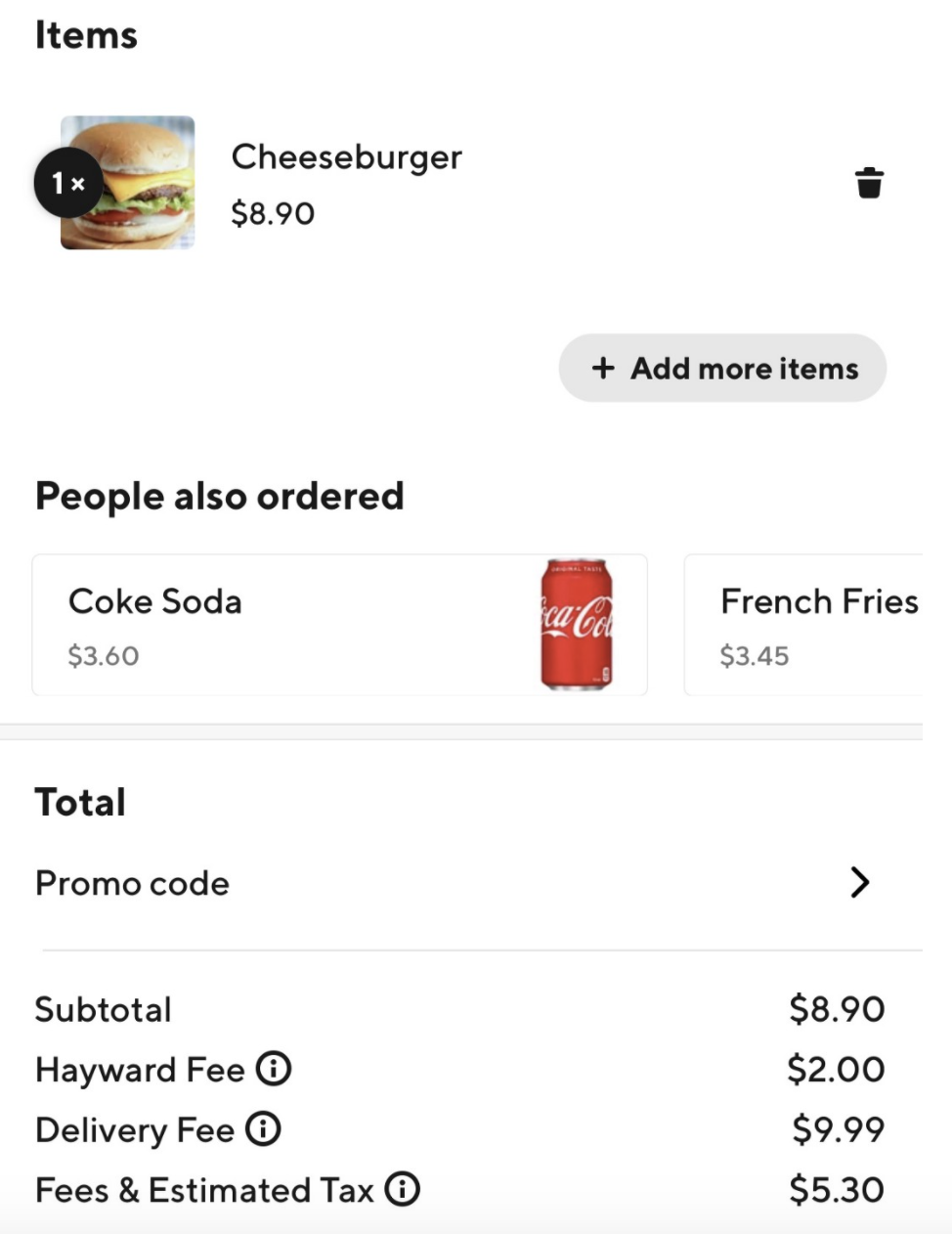Screenshot Description:

The background of the screenshot is white. 

In the upper left-hand corner, the word "Items" is displayed in bold black text. Approximately two lines below that, there is a small square featuring an image of a cheeseburger. Extending slightly off the left edge is a black circle with the number "1" in white text, followed by a small "X" to the right. 

To the right of the cheeseburger image, the word "Cheeseburger" is written in bold black text. Two lines below the word "Cheeseburger," the price "$8.90" is shown. Further to the right, there is a black trash can icon. 

Approximately three lines down from the trash can icon, on the right side, there is a gray oval containing a plus sign and the phrase "Add more items" in bold black text. 

Approximately three lines below the "Add more items" button, the phrase "People also ordered" appears in bold black text on the left. About two lines below that, there is a rectangle outlined in gray. 

Within this rectangle, on the left side, "Coke soda" is written in black, with "$3.60" displayed underneath. To the right, there is an image of a Coca-Cola can. To the right of this image, a partially visible outlined rectangle contains the text "French fries" with "$3.45" shown below it.

A gray horizontal line runs across the screen, separating the sections. Below this line, on the left side, the word "Total" is displayed in bold black text. About two lines down, there is the phrase "Promo code," aligned to the left, with a right-pointing arrow on the right side of this line. 

Another light gray horizontal line appears below the "Promo code" line. Beneath this line, the word "Subtotal" is shown on the left, with "$8.90" displayed on the right.

Further below, "Hayward fee" is listed with an information icon (a circle with an "i" in the center) and is priced at "$2.00."

"Delivery fee" is listed next, also accompanied by an information icon, and priced at "$9.99."

Below that, the section labeled "Fees & estimated tax" includes another information icon, with the amount "$5.30" listed beside it.